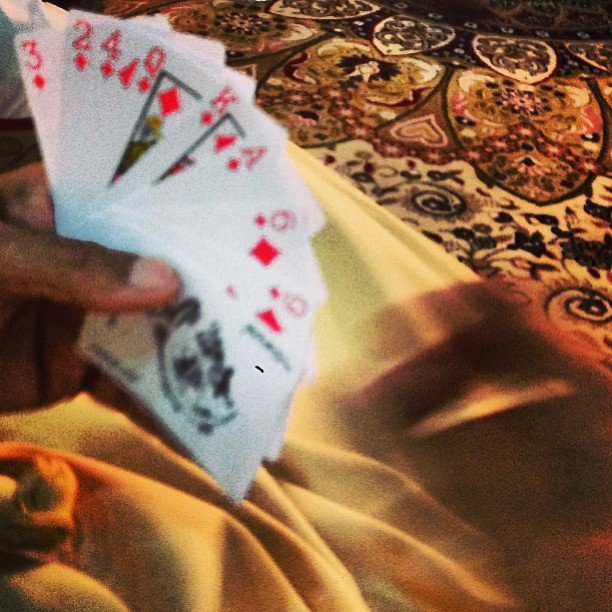A dimly lit, indoor color photograph captures an intimate scene with a slightly grainy and out-of-focus aesthetic. The focal point of the image lies just left of center, where an African-American hand emerges from the left edge, displaying a fanned-out arrangement of nine playing cards. The cards, arranged from top to center in the hand, are: the Three of Diamonds, Two of Diamonds, Four of Clubs, Queen of Diamonds, King of Diamonds, Ace of Diamonds, Six of Diamonds, Nine of Diamonds, and a Joker.

In the background, a crumpled yellow blanket spreads across the lower portion of the frame, predominantly in the left corner. In the upper right corner, a portion of a yellow and dark green oriental rug is visible. The rug features a quarter of a circular, ornate pattern that subtly enriches the background. The lower right corner of the photograph is noticeably darker, adding to the image's overall moody and dim atmosphere. Despite the photograph's graininess and blurred focus, the textured backdrop and the array of playing cards create a compelling visual narrative.